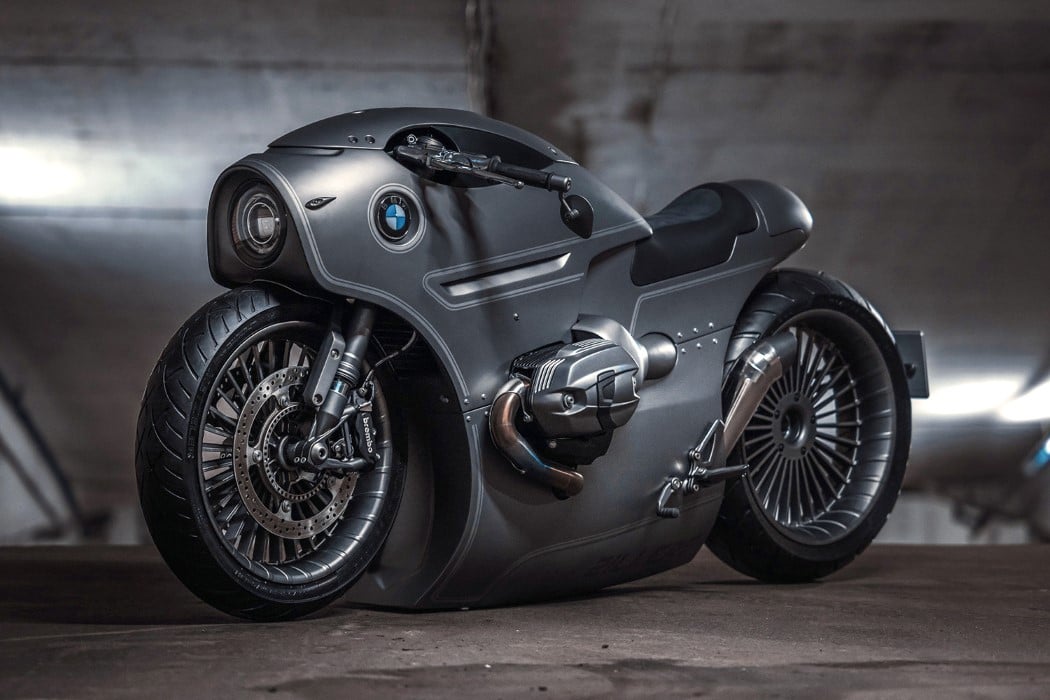The image captures a sleek, futuristic BMW motorcycle set against a gray concrete background, likely inside a garage given the hanging lights visible in the scene. The motorcycle boasts a streamlined, high-tech design with an all-black or dark gray chrome finish. Its two black, slick tires contrast with the metallic body that encases much of the mechanical parts. A circular BMW emblem is prominently displayed above the front wheel. The design features a higher hump at the top that tapers down, along with a singular circular headlight at the forefront. The handlebars protrude from either side above a metal cover where traditional motorcycle steering would be. The seat appears to be black leather, designed for the rider to lean forward, mimicking the riding style of a superhero like Batman. The bike's engine is partially exposed, adding to its souped-up, futuristic aesthetic.